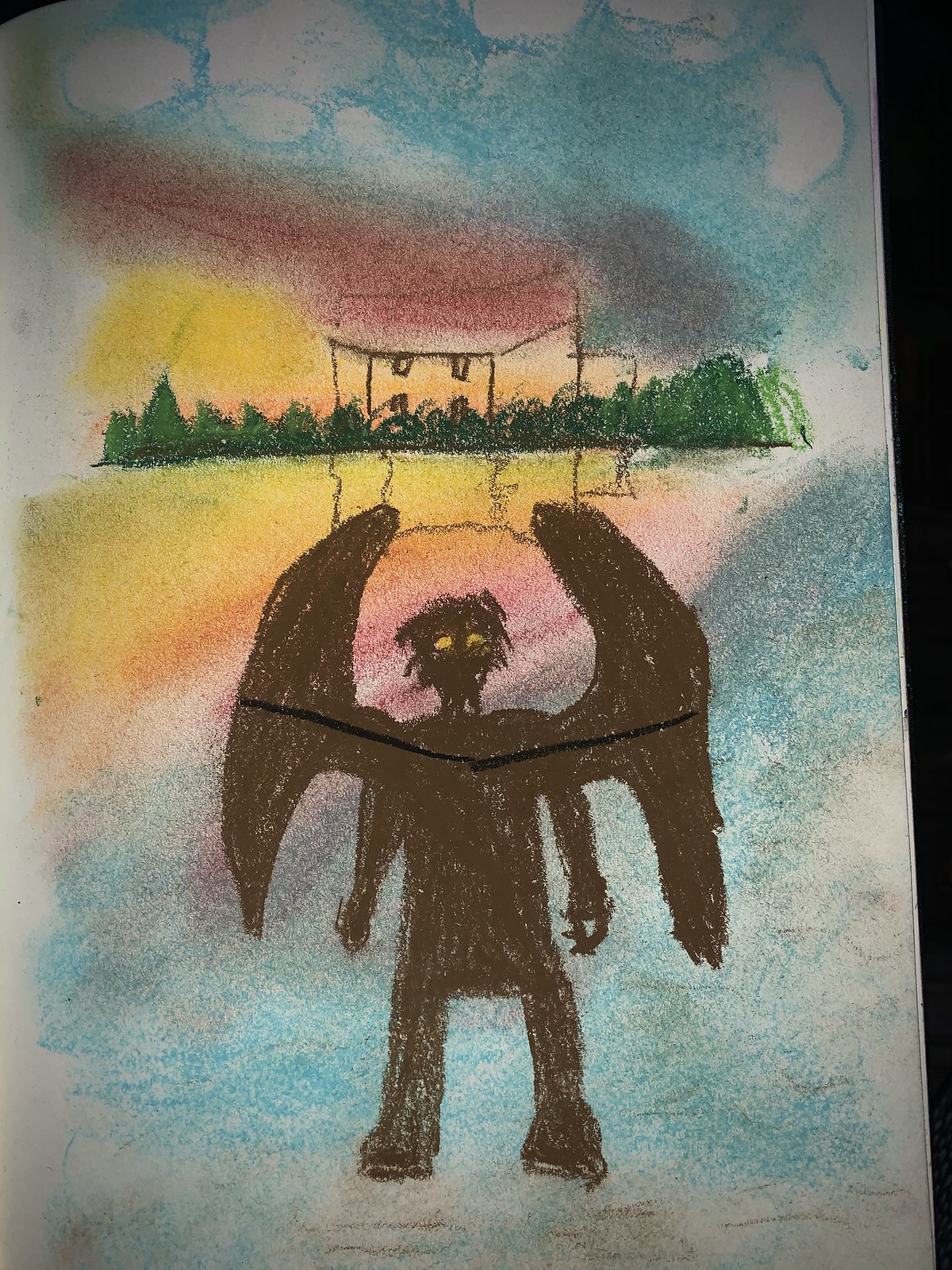A child’s drawing is depicted on white paper, adorned with a spectrum of pastel colors – blue, pink, and yellow – messily shaded across the background. At the top, the sky is blue with fluffy white clouds, where the white is just the paper showing through. Below the sky, a sunset or sunrise is hinted at with patches of yellow. To the far back, a rudimentary pencil drawing of a house, constructed with simple lines and squares for windows, stands behind a row of green bushes and distant trees. The house’s reflection in front of it is notably shaded with yellow and red, creating a mirrored effect on a supposed body of water. Dominating the foreground is the striking image of an ambiguously dark figure that seems to straddle the line between angelic and demonic. This figure, fully colored in brown or black, stands with wide-spanned wings, hauntingly white or glowing yellow eyes, scraggly hair, and a bold black line slicing across its form from one wing to the other. The overall composition evokes a gothic, eerie atmosphere, atypical of typical children’s drawings.